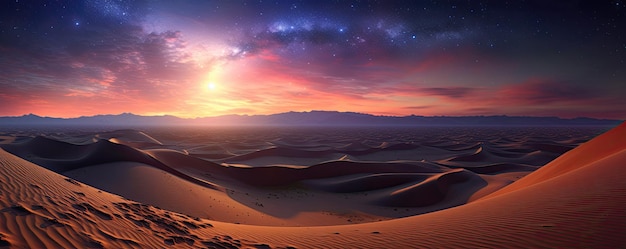The image portrays a stunning and highly stylized desert landscape, potentially a hyper-realistic artificial intelligence creation or heavily retouched photograph. Dominating the foreground are reddish-orange sand dunes bathed in the warm hues of a setting sun. The dunes look like rolling hills of sand, stretching into the background where shadowy mountain ranges can be faintly seen. The vibrant sunset sky transitions from brilliant yellows, oranges, and reds near the horizon to deep navy blues and blacks higher up. Stars, tinged with a bluish hue, twinkle in the upper reaches of the sky, adding a cosmic feel to the scene. Shadows cast by the undulating dunes accentuate the mysterious and awe-inspiring atmosphere. The sun's position creates a dramatic lighting effect, illuminating one particular area of the sky through a break in the clouds, suggesting an ethereal and otherworldly setting. The color palette includes violent purples, maroons, blacks, and browns, enhancing the image's surreal and captivating quality.